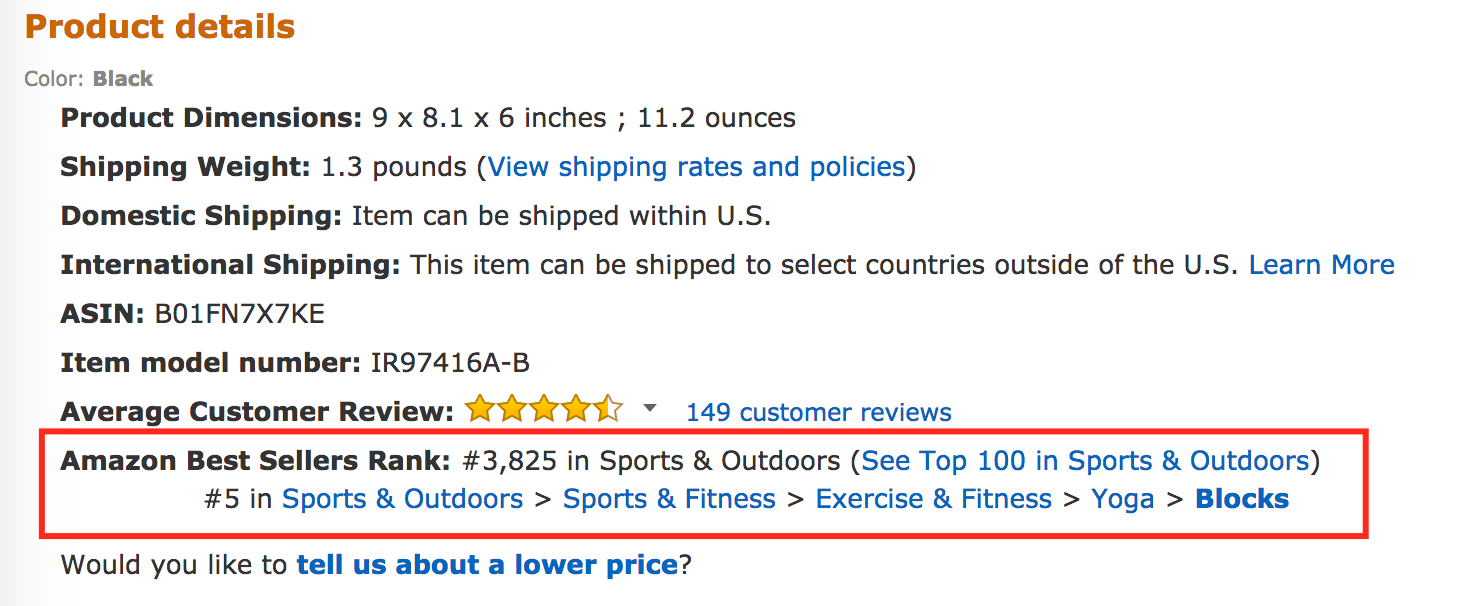**Caption:**

The image displays a detailed product information section set against a light gray background. In the upper left corner, there is a bold, orange heading that reads "Product Details." Below this, in gray text, it mentions "Color: Black," despite the font being gray. Further down, in black text, it lists "Product Dimensions: 9 x 8.1 x 6 inches; 11.2 ounces."

The next line in bold black text states "Shipping Weight:," followed by "1.3 pounds" in regular black text, with a parenthesis in blue indicating "View shipping rates and policies" for domestic shipping. It also mentions that the item can be returned within the U.S. For international shipping, it says in bold black, "International Shipping:" and then in regular text, "This item can be shipped to select countries outside the U.S.," with "Learn more" in blue.

Following this, the image provides the ASIN (Amazon Standard Identification Number) in capital letters as "ASIN: B01N7X7KE." Next, in bold, it mentions "Item Model Number:," specified as "IR97416AB" in uppercase. 

In bold black text, it highlights "Average Customer Review," showing approximately four and a half stars, followed by "149 customer reviews" in blue.

Encased in a red box, the image includes the "Amazon Best Sellers Rank" with a rank of "#3,825 in Sports and Outdoors," and in blue, it says "(See Top 100 in Sports & Outdoors)." Additionally, it lists "#5" in Sports and Outdoors subcategories with black arrows pointing to subsequent categories: "Sports & Outdoors" -> "Exercise & Fitness" -> "Yoga" -> "Blocks."